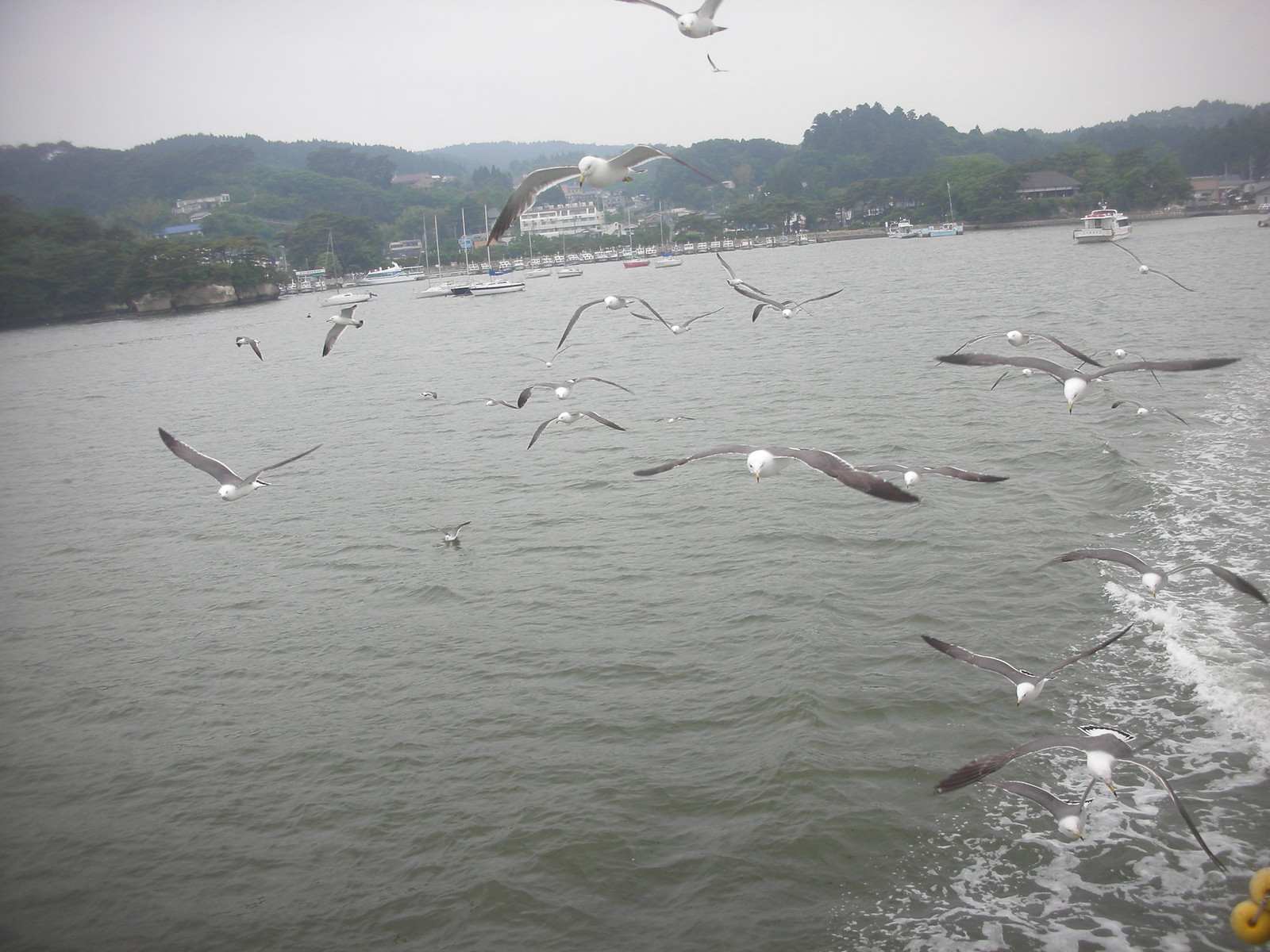The photograph captures a small flock of gulls with white heads and dark gray bodies, their wings darker near the tips, flying low over the relatively calm, gray water. Most of the gulls are moving towards the photographer. In the lower right-hand corner, the boat from which the photo is taken creates a visible wake, alongside two small yellow floats. The backdrop features a variety of boats, including several moored sailboats and a powerboat traveling away from the camera. On the far side of the water, rolling hills adorned with trees frame the scene, and amidst the greenery, various low-rise buildings are visible, including what appears to be a hotel. The overall ambiance suggests an overcast day, adding a muted light to the serene maritime setting.